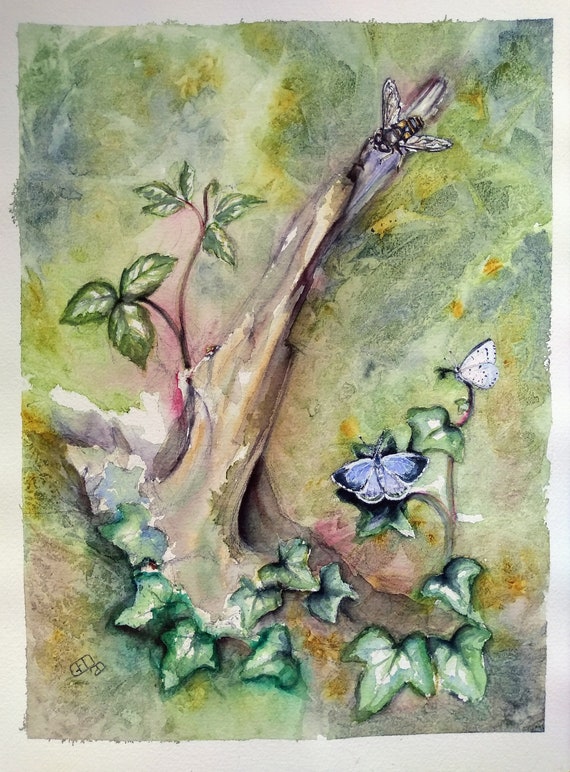The image is a watercolor painting depicting an outdoor scene with a broken tree trunk at the center. The background features varying shades of green and yellow, creating a natural and serene ambiance. The broken tree trunk, centrally positioned, has new life springing from it with two thin branches on the left side adorned with green leaves. On the right, two butterflies rest on additional green foliage – a blue butterfly is situated closer to the middle of the image, while a white butterfly perches higher up. A fly hovers near the top of the tree trunk, adding to the sense of ongoing life and movement. Scattered on the ground before the trunk are multiple green leaves. The carefully applied watercolors enhance the ethereal quality of the scene, and the image is framed by a plain white border.